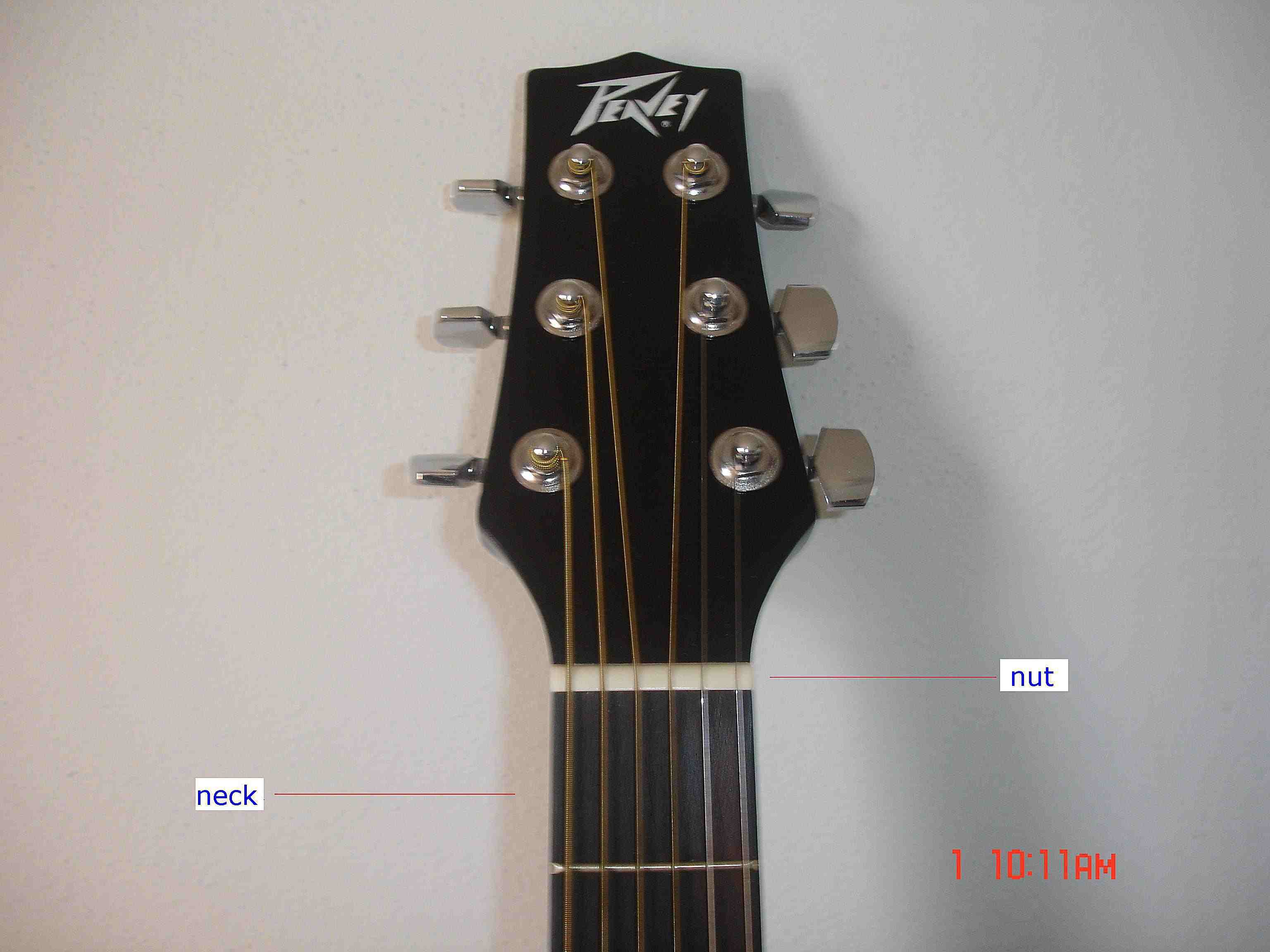The image depicts the upper section of a black Peavey guitar, specifically showcasing the headstock and tuning pegs. The guitar leans against a white wall, casting shadows to the right and behind the neck. The headstock features a brand logo in stylized white letters reading "Peavey." The tuning knobs and yellow strings extend from the headstock down the neck. A white nut sits at the junction between the headstock and neck. On the left side of the image, a blue-labeled rectangle with a red line points to the guitar's neck, while a similar rectangle on the right side points to the nut. In the bottom right corner, a time stamp in orange font reads "1:10:11 a.m."